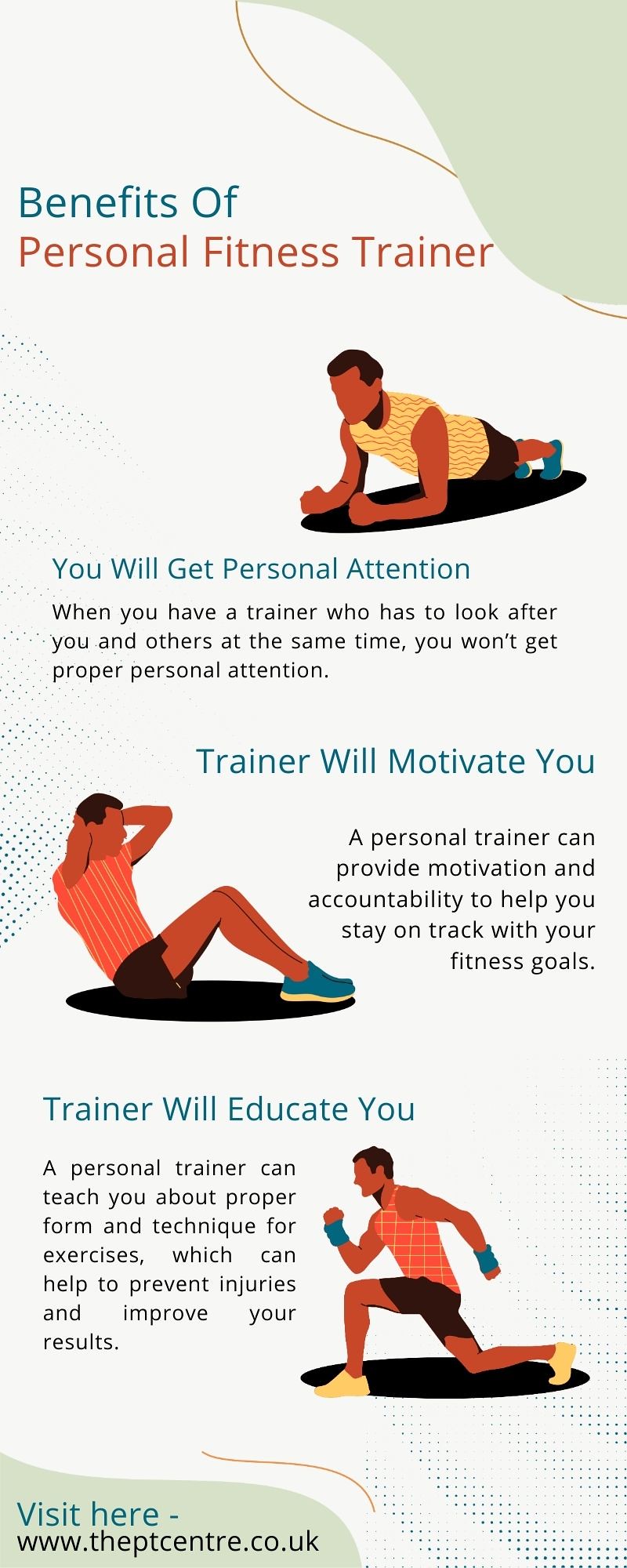The image features a visually appealing poster titled "Benefits of a Personal Fitness Trainer," prominently displaying information underscored by vibrant colors such as tan, blue, orange, green, yellow, black, and white. The poster occupies the entire frame of the image, suggesting it is an advertisement likely found at a gym or a related fitness setting.

The poster outlines three key benefits of having a personal fitness trainer:

1. **Personal Attention:** The poster emphasizes that with a personal trainer, individuals receive focused attention, as opposed to trainers who must divide their time among multiple clients.
   
2. **Motivation and Accountability:** It highlights the motivational support and accountability a personal trainer provides to keep clients aligned with their fitness goals.
   
3. **Education on Proper Form and Technique:** It states that a personal trainer can educate clients on correct exercise form and technique, which is crucial for preventing injuries and enhancing workout results.

Additionally, the poster includes a call-to-action at the bottom, directing viewers to "www.thePTcenter.co.uk" for more information. The design is augmented by computer-generated illustrations depicting characters performing various exercises. The overall aesthetic suggests a modern, app-like interface, reinforcing its suitability for tech-savvy gym-goers.